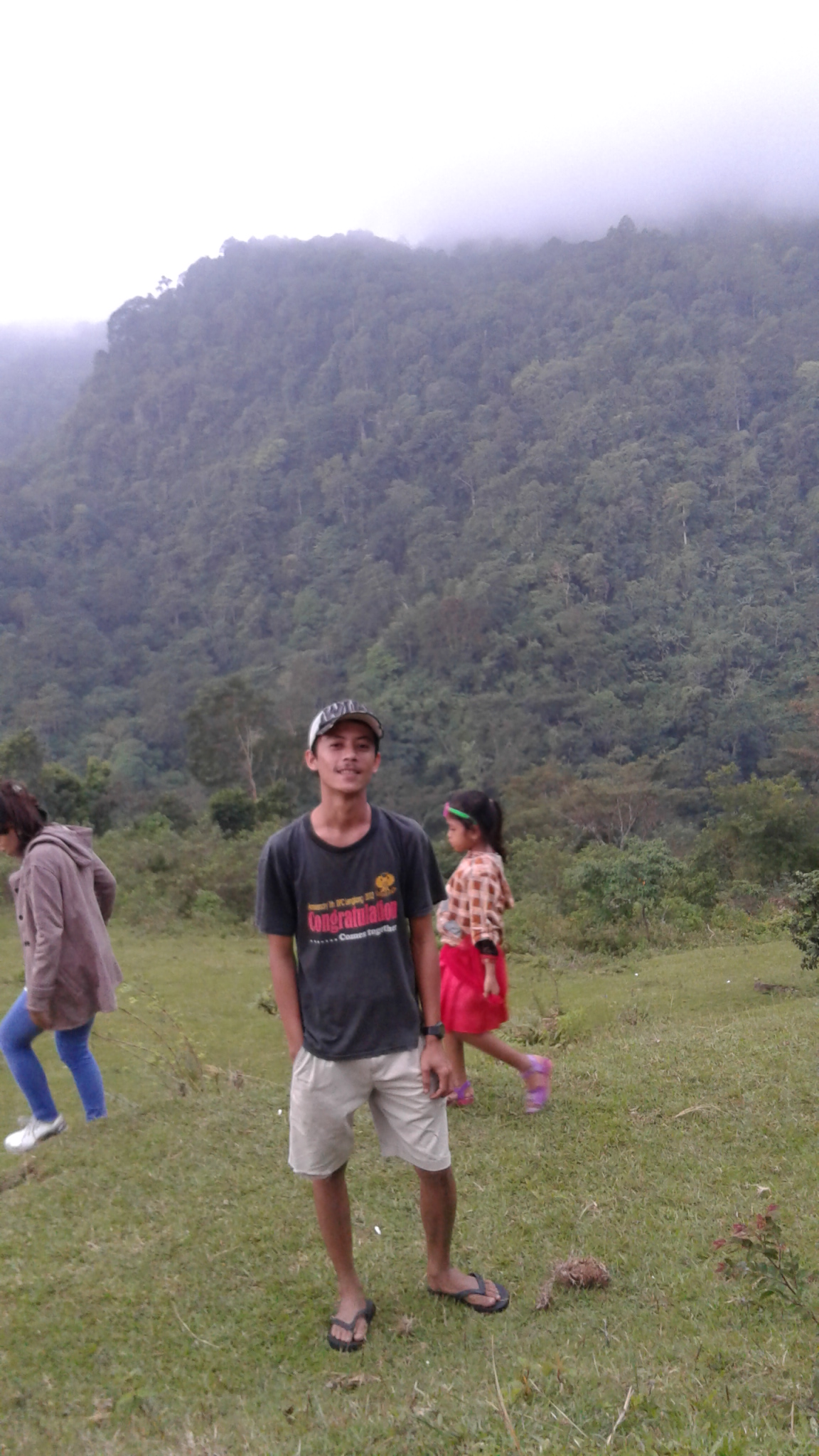In this photograph taken outdoors on a grassy hillside, three people are prominently featured against a backdrop of a vast, tree-covered mountain or cliffside, partially veiled in distant fog and under a bright yet grey and foggy sky. 

At the center forefront stands a tanned-skinned individual wearing a black graphic short-sleeve T-shirt with red lettering that reads "Congratulations" and white writing underneath that says "Comes Together." They are dressed in white shorts, black sandals, and a black and white baseball cap. Behind this person to the left, a person partially cropped out by the image's edge wears a gray-colored, open button-up hoodie jacket, blue jeans, and white shoes. The top part of this person's head is not visible. Directly behind the central figure and to the right stands a young girl with light brown skin and dark brown hair, adorned with a green and pink headband. She is dressed in a brown and white plaid long-sleeve shirt, a pink skirt, and pink sandals. The scene exudes a serene, natural ambiance, blending the calmness of the foggy, wooded mountain with the casual, everyday attire of the individuals captured.